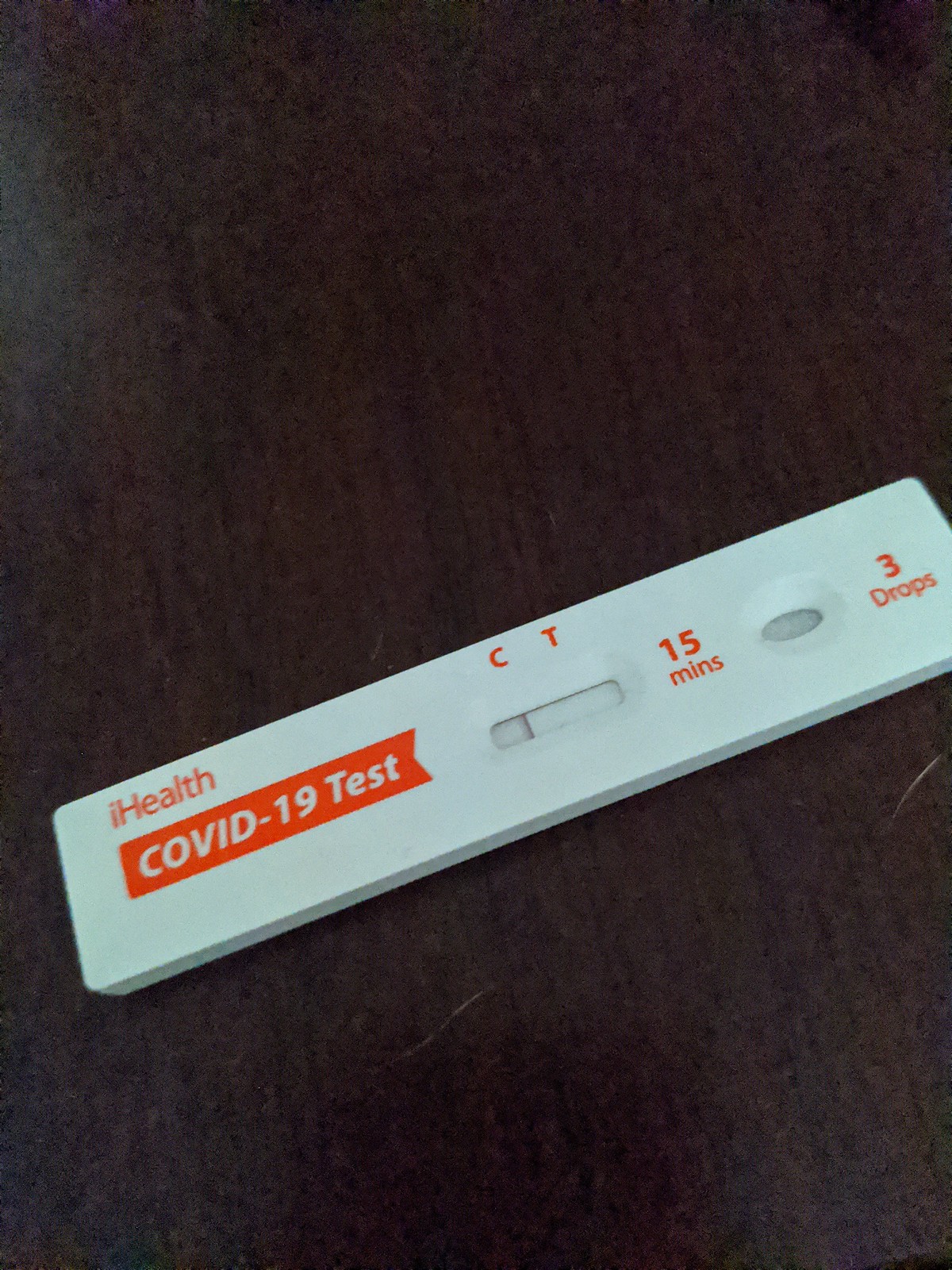A detailed color photograph captures a COVID-19 test situated diagonally on a dark surface. The test, a long white rectangular device, prominently features several markings and texts. On the left side, it reads "iHealth" with the text in lowercase. Below this, an orange banner displays "COVID-19 Test" in white letters. To the right, there is a rectangular window labeled with "C" and "T" in orange letters, indicating the control and test lines. A thin vertical line is visible beneath the "C" marker. Further right, the test shows the inscription "15 mins," with "mins" abbreviated. Adjacent to this is a small oval window, accompanied by the instruction "3 drops" on its right. This image is oriented vertically, being taller than it is wide, and contains no people, animals, plants, signs, buildings, mechanical objects, or vehicles, focusing solely on the COVID-19 test.